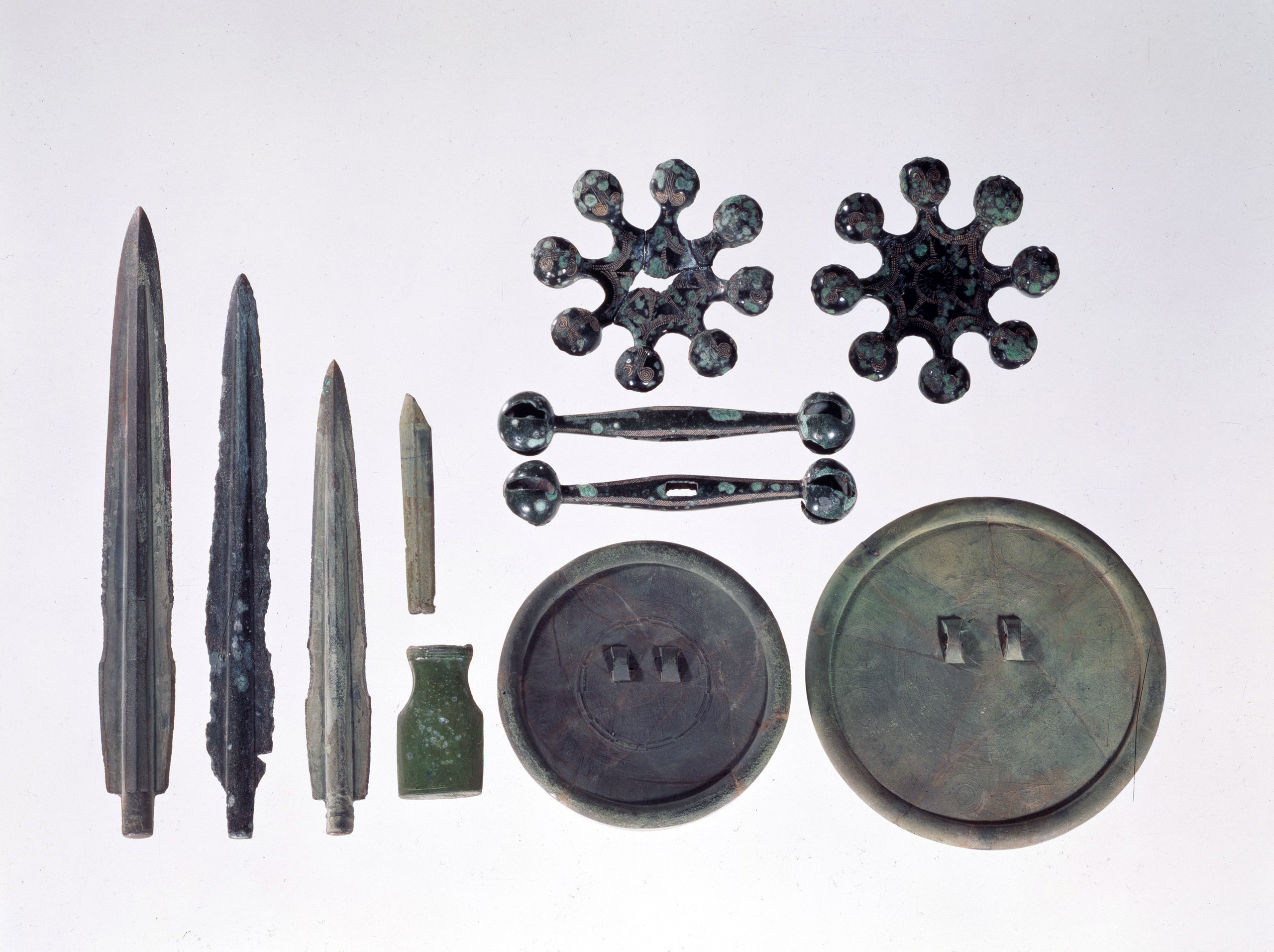This close-up image showcases an array of ancient Anglo-Saxon style artifacts displayed on a completely white background. On the very left, there are four different-sized, dagger-like stone tools without handles, each varying in height, with the tallest to the left and the shortest on the right. The second object from the left is darker in color, closer to black, in contrast to the grayish hue of the others. To the right of these blades is a small fragment resembling the top part of one of these knives, positioned above a greenish jar.

Further right are two circular objects resembling shields, viewed from the back, with visible arm straps indicating how they would be held. Above these shields, the image reveals two elongated metal rods with ball-like ends, reminiscent of dumbbells. The lower rod features a small rectangular opening in its center. 

At the top-right section of the image, there are two star-shaped metal objects, possibly belt clasps. Their distinctive shape includes protruding rounded elements at the ends of each ray, which slightly resemble the form of a flattened jack. The overall collection of artifacts appears weathered and possibly rusted, indicative of their ancient origins.